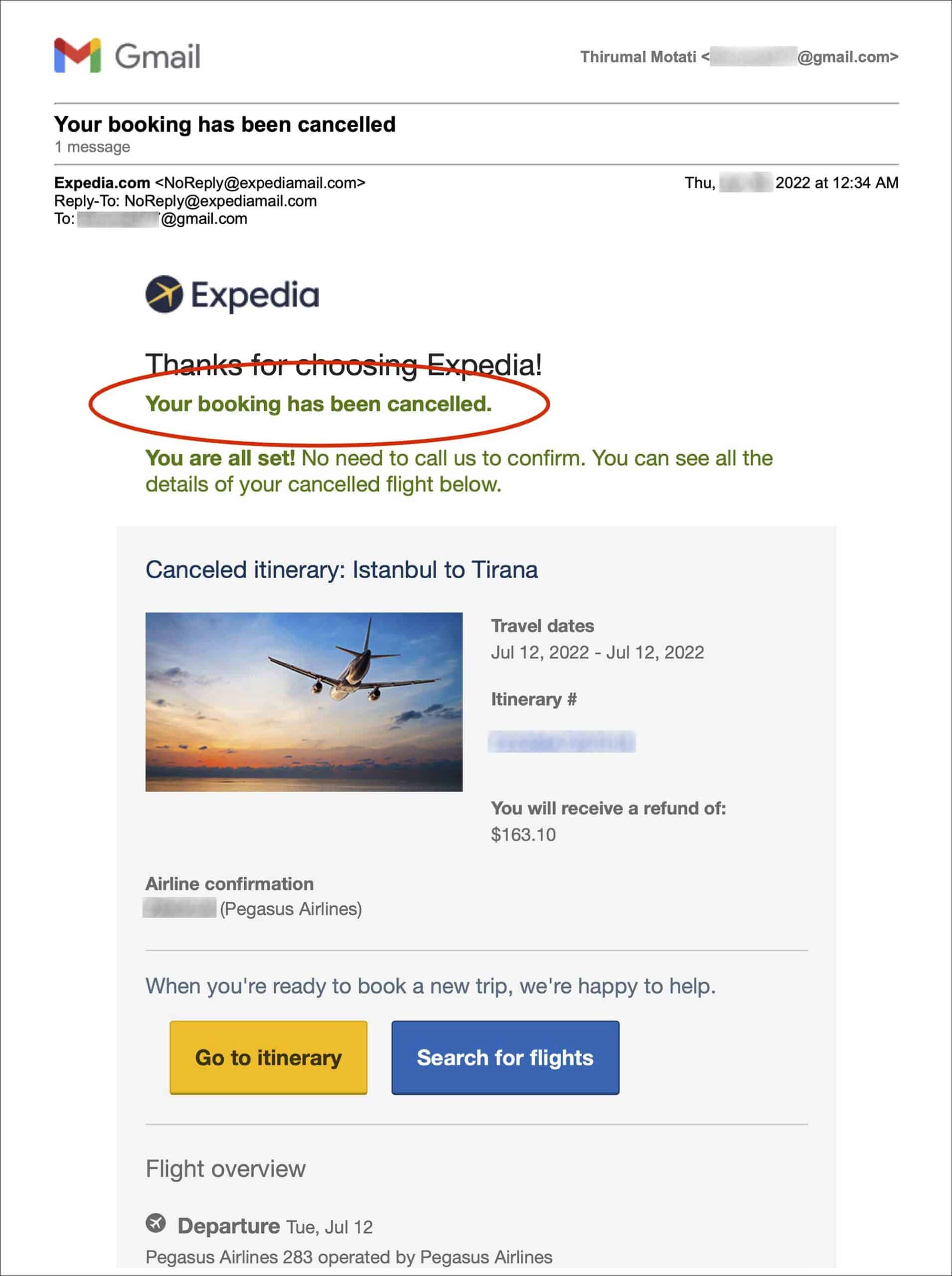The image is a screenshot from the Gmail mobile application, identifiable by its tall rectangular proportions. At the top of the interface, the Gmail logo is prominently displayed, featuring an 'M' in Google's signature colors of blue, red, yellow, and green, accompanied by the text "Gmail." Directly beneath this header, a notification states in bold text, "Your booking has been canceled" with a subtext indicating "1 message."

The sender information follows, identified as "Expedia.com" with the email address "no-reply@expediamail.com," and the recipient's email address is partially visible but blurred out for privacy.

The body of the email is dominated by the Expedia logo, a black circle featuring a yellow airplane. The message begins with "Expedia" followed by a thank-you note: "Thank you for choosing Expedia." The critical information "Your booking has been canceled" is highlighted with a red circle, ensuring it stands out. Further text reassures the recipient: "You're all set. No need to call us to confirm. You can see all the details of your canceled flight below."

Adding to the visual details is a large gray box containing an image of a plane flying into the sunset. Supplementing this visual cue, the text confirms, "You will receive a refund of $163.10 on Pegasus Airlines."